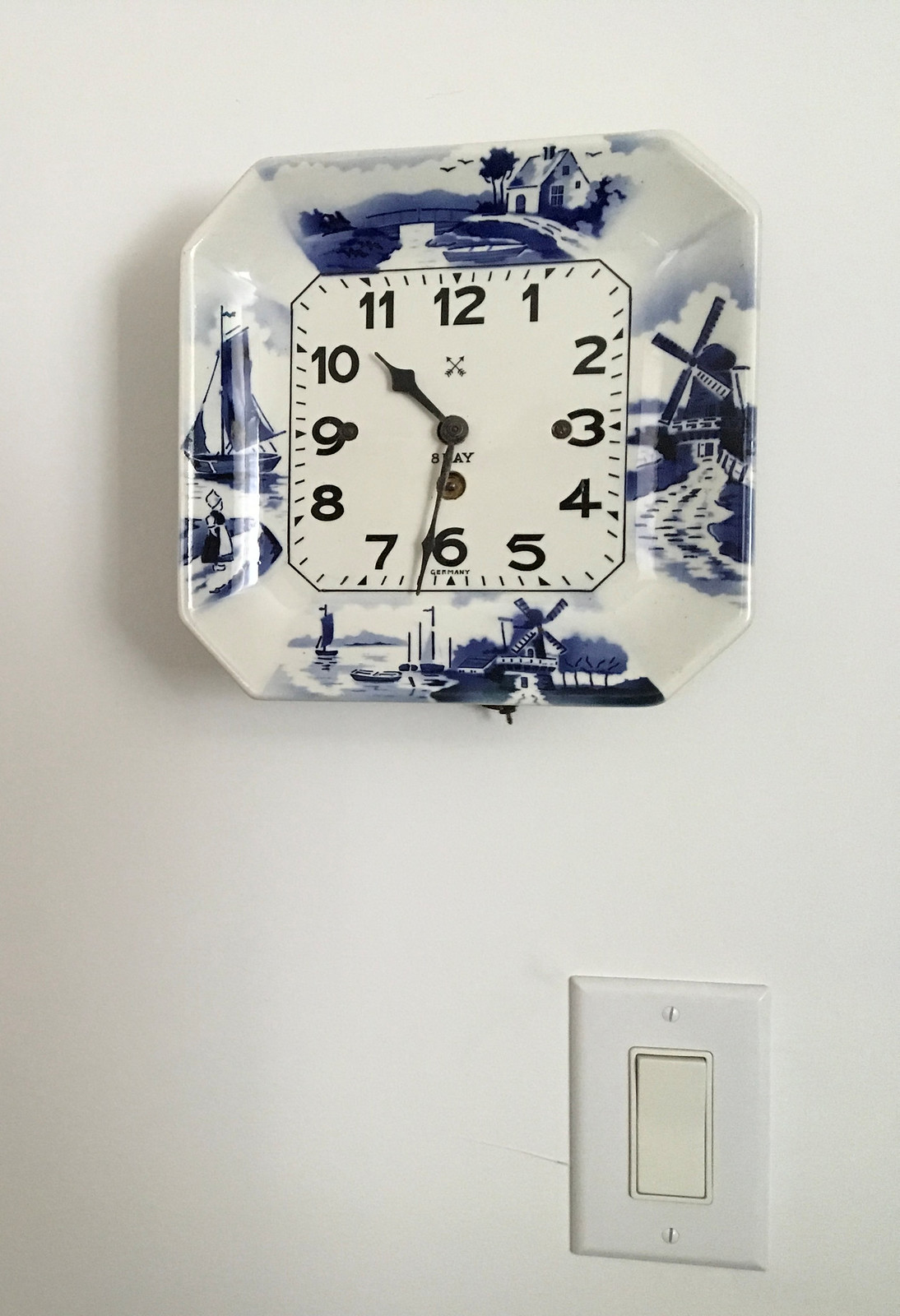This image features a detailed clock hanging on a bright white wall. The clock, resembling a dinner plate in its overall shape—though it is actually octagonal—showcases intricate Delft blue designs at strategic points: the top, bottom, left, and right. At the top, a house stands beside a canal, surrounded by birds and trees. The bottom and right sections are adorned with images of windmills and bodies of water, while the left side depicts a girl in traditional Dutch clothing alongside a sailboat. The clock's center has a white background, upon which black numbers are painted, with black metal clock hands—one long for minutes and one short for hours—indicating the time as approximately 10:32. The middle of the clockface includes partially visible letters, seemingly forming the word "S?AY." Directly beneath the clock, there is a white, standard light switch with a matching cover plate, secured by screws at the top and bottom, enhancing the pristine, monochromatic theme of the wall.